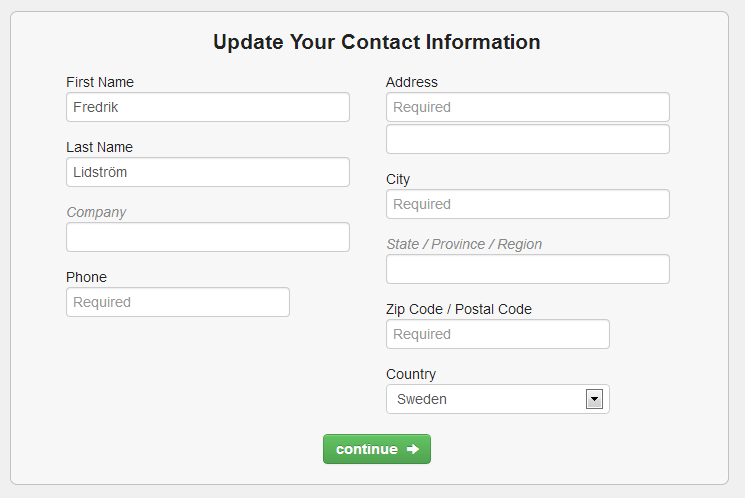The image is a screenshot with a gray background. Dominating the screen, there is a large, slightly lighter gray square. At the top of this square, bold black text reads "Update Your Contact Information."

Below the title, the screen is divided into two columns filled with form fields. The left column includes four fields: 
1. **First Name:** Inside the white rectangular box is the name "Frederick," spelled out as "F-R-E-D-R-I-K."
2. **Last Name:** The box contains the name "Lidstrom."
3. **Company:** The label is gray, indicating optionality.
4. **Phone:** The box is labeled "required," hinting it must be filled out.

The right column focuses on the address and includes five fields:
1. **Address Line 1:** The box is labeled "required" in gray.
2. **City:** Another box labeled "required" in gray.
3. **State/Province/Region:** This field is also labeled in gray.
4. **Zip/Postal Code:** The label is in black with "required" indicated inside the box in gray.
5. **Country:** The box contains the word "Sweden" and features a drop-down arrow to select the country, situated on the right side of the box.

Centered at the bottom of the square is a green rectangular button that reads "Continue" in white, accompanied by a right-pointing arrow.